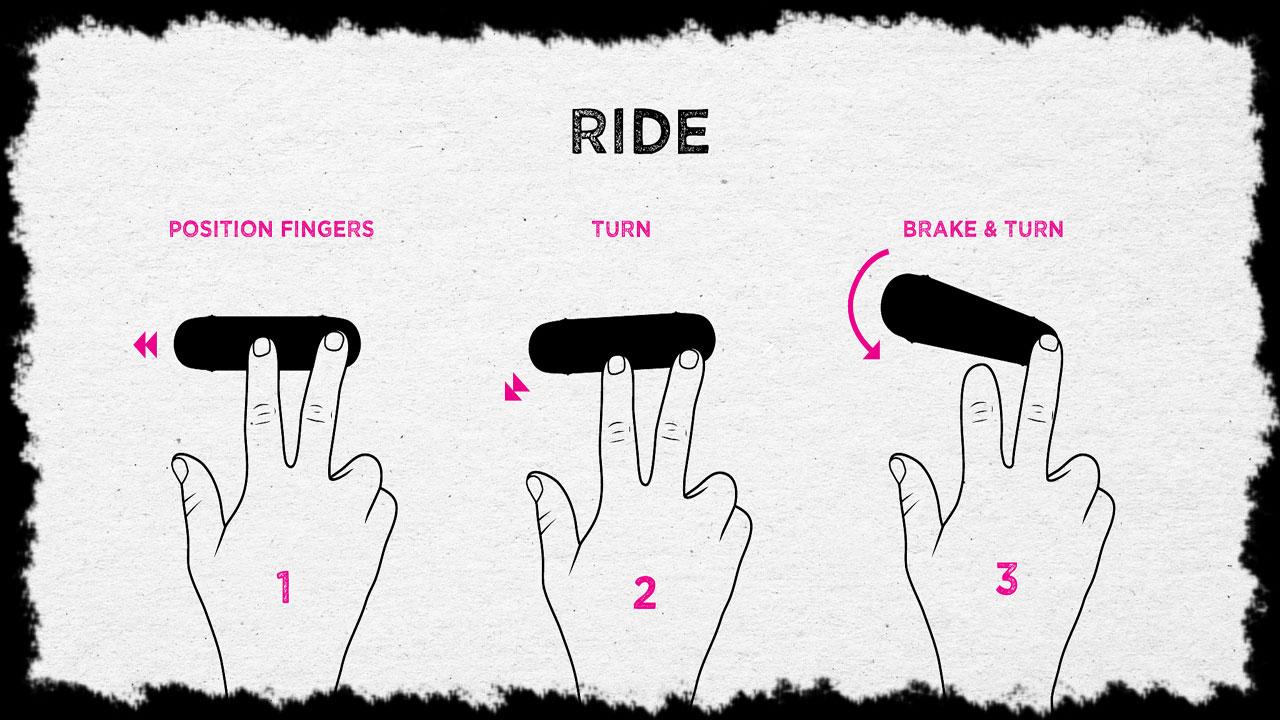This horizontally aligned rectangular image features a hand-drawn design on a white background with a rough, irregular black border. At the top center, the word "RIDE" is displayed in bold black uppercase letters. Below "RIDE," there are three titling labels in pink: "Position Fingers," "Turn," and "Break and Turn." Each title corresponds to one of three hand-drawn illustrations of hands numbered from one to three in pink.

- The left illustration, labeled "Position Fingers," shows two fingers touching a black oval shape with pink arrows pointing left.
- The middle illustration, labeled "Turn," shows two fingers again, with a black oval shape and pink arrows pointing diagonally to the bottom left.
- The right illustration, labeled "Break and Turn," depicts a single middle finger touching a black oval shape and an arrow curving to the right.

Each hand interaction likely serves to instruct viewers on the sequence and method for positioning, turning, and breaking and turning the object represented by the black oval shapes.